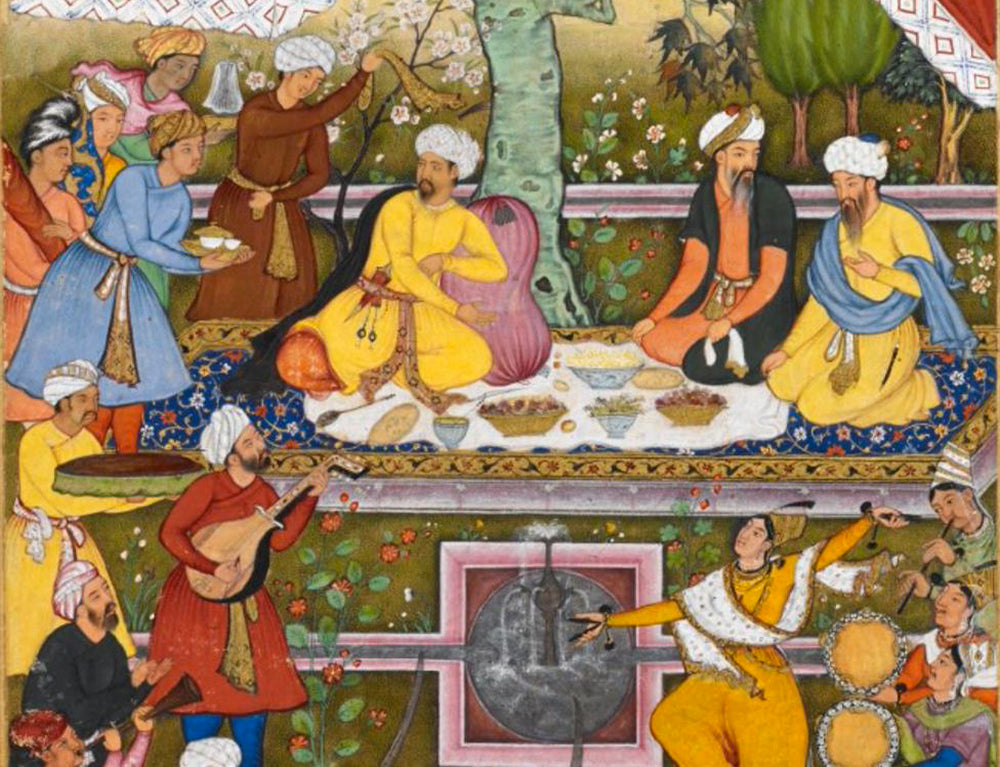This intricate and historic painting, likely of an oriental or possibly Hindi origin, vividly captures a festive and ornate scene. The lower portion of the image showcases a lively musical and dance performance. At the center, a female dancer in a yellow outfit, adorned with a white scarf and a hat, gracefully moves. Surrounding her are female musicians; one plays a flute while others handle drums. Male musicians on the left, dressed in colorful tunics and scarves, play a variety of instruments including a lute and a horn. Other details include a central fountain that resembles a goblet with water cascading, set against a backdrop of green leaves and orange flowers.

Above this lively scene, the upper section depicts an elegant picnic setting on a white layer of material. Three men, dressed in vibrant robes of yellow, blue, and orange, and wearing turbans, are seated around an abundant feast of various cups and baskets of food. One of the men reclines against a cushion near a tree, while two others seem to be engaged in conversation. To the far left, several servants, also clad in colorful robes but with different head attire, attend to the seated men by offering food, drink, and comfort such as waving a piece of material above their heads. Ornamental trees and flowers embellish the distant background, adding to the overall opulence and specificity of the scene's period. The image bursts with color, featuring primarily yellow, blue, green, with splashes of pink, brown, gold, and orange, providing a detailed snapshot of a celebratory moment rich in cultural history.